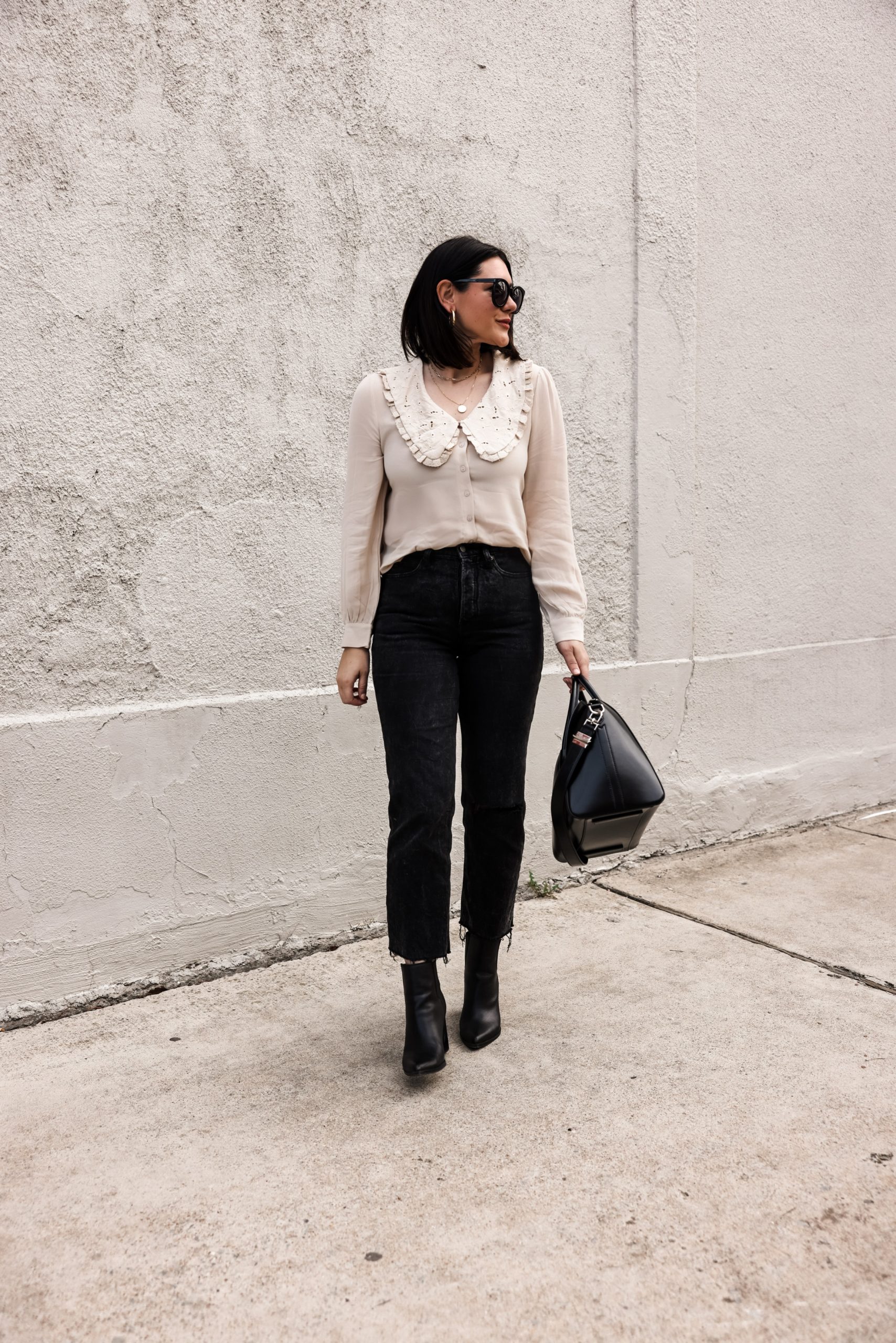In a fashion photograph set against an urban backdrop, a woman in her 30s stands confidently in front of a textured white stucco wall. She is framed from head to toe, positioned centrally on a paved sidewalk with a concrete floor. The image captures her from the front, though she turns her head to her right, offering a captivating profile. Her black hair, styled to brush back from her forehead and loop behind her ear, extends just past her neckline. 

She sports dark oversized sunglasses and hoop earrings, adding a touch of glamour. Her outfit pairs contrasting elements: a white long-sleeve sweater with a lace neckline and a scooped collar, matched with black pants that end just above her black high-heeled ankle boots. Completing her ensemble, she carries a large black leather handbag with her left hand resting by her side. The photograph, steeped in tones of off-white and black, exudes a minimalist yet chic vibe typical of fashion photography, likely ideal for promoting the stylish ensemble.